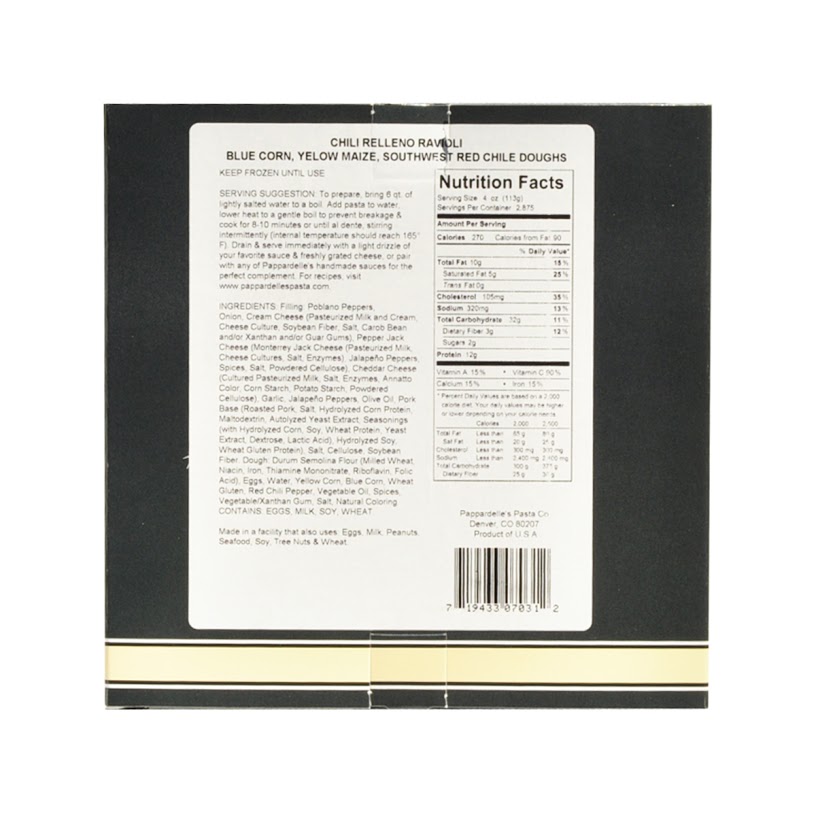Color Photograph: Back of Chili Relleno Ravioli Box

In this color photograph, we are presented with the backside of a package for Chili Relleno Ravioli, prominently packaged in a sleek black box adorned with a horizontal yellow stripe at the bottom. At the center of the box is the black and white nutrition label.

The text on the package reads: "Chili Relleno Ravioli. Blue corn, yellow maize, southwest red chili doughs. Keep frozen until use. Serving suggestion."

Preparation instructions are detailed as follows:
1. Bring six quarts of lightly salted water to a boil.
2. Add the pasta to the water.
3. Lower heat to a gentle boil to prevent breakage.
4. Cook for eight to ten minutes or until al dente, stirring intermittently.
5. Ensure the internal temperature reaches 165 degrees Fahrenheit.
6. Drain and serve immediately with a drizzle of your favorite sauce and freshly grated cheese or complement with any of Pappardelle's handmade sauces.

The box also provides a website for additional recipes: www.pappardellespasta.com.

The ingredients list for the filling includes: poblano peppers, onion, cream cheese (pasteurized milk and cream, cheese culture, soybean fiber, salt, carob bean gum/xanthan gum/guar gum), pepper jack cheese, Monterey Jack cheese (pasteurized milk, cheese culture, salt, enzymes), jalapeno peppers, spices, powdered cellulose, cheddar cheese (culture, pasteurized milk, salt, enzymes, annatto color), cornstarch, potato starch, garlic, jalapeno peppers, olive oil, pork base (roasted pork, salt, hydrolyzed corn protein, maltodextrin, autolyzed yeast extract, seasonings with hydrolyzed corn/soy/wheat protein, yeast extract, dextrose, lactic acid, hydrolyzed soy/wheat gluten protein, salt, cellulose, soybean fiber).

The dough is made of durum semolina flour, milled wheat (niacin, iron, thiamine mononitrate, riboflavin, folic acid), eggs, water, yellow corn, blue corn, wheat gluten, red chili pepper, vegetable oil, spices, vegetable/xanthan gum, salt, natural coloring. Note that the product contains eggs, milk, soy, and wheat, and is made in a facility that also processes eggs, milk, peanuts, seafood, soy, tree nuts, and wheat.

The nutrition facts are as follows:
- Serving size: 4 ounces
- Servings per container: 2.875
- Calories: 270
- Calories from fat: 90
- Total fat: 10 grams
- Saturated fat: 5 grams
- Trans fat: 0 grams
- Cholesterol: 105 milligrams
- Sodium: 320 milligrams
- Total carbohydrate: 32 grams
- Dietary fiber: 3 grams
- Sugars: 2 grams
- Protein: 12 grams
- Vitamin A: 15%
- Vitamin C: 90%
- Calcium: 15%
- Iron: 15%

This photograph offers a comprehensive glimpse of the product’s packaging, ingredients, preparation instructions, and nutritional information.